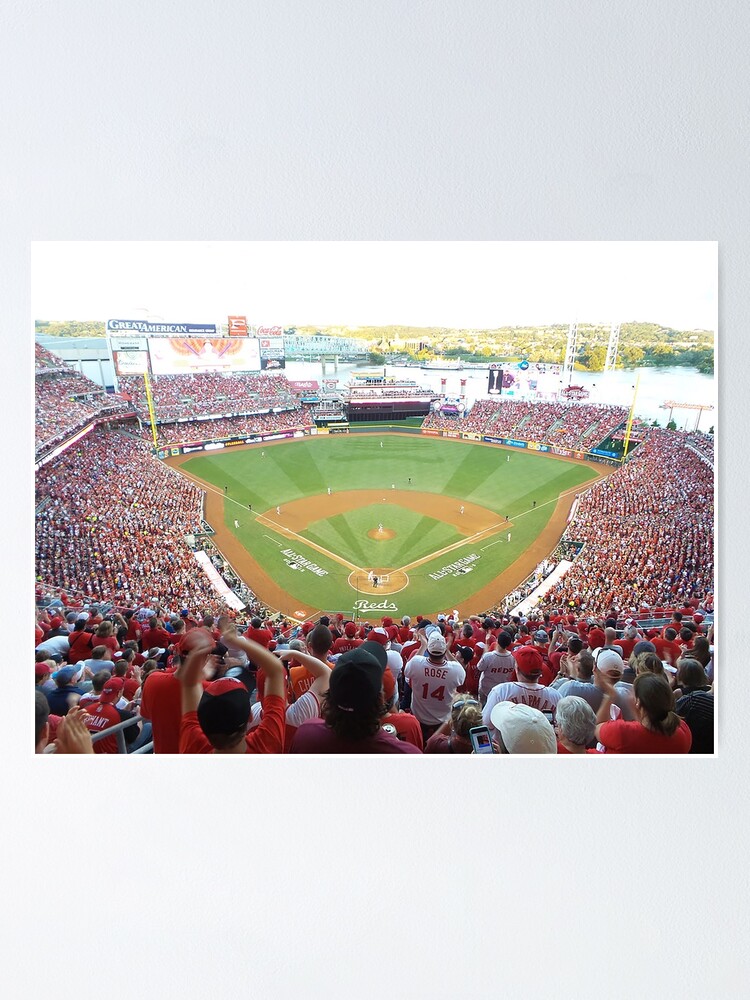The image captures a panoramic view of a vibrant baseball game taking place in a large stadium in the United States. From our vantage point high up in the bleachers behind the pitcher's mound, we look out over the entire field, with the bases arranged in a diamond pattern: first base to the right, second and third bases farther away, and home plate directly in front. The lush, well-maintained pitch features striped patterns of dark and light green grass, punctuated by a light brown cut-out area at the center of the diamond, indicating active play. The stadium is packed with enthusiastic supporters, predominantly wearing red and white, suggesting a strong presence of fans for the Cincinnati Reds, further confirmed by the large "Reds" lettering visible on the field. The clear sky above casts a white light over the scene, and beyond the bustling stadium lie tranquil, green hills. TV screens and monitors typical of professional stadiums are visible, and the fans in the foreground, many wearing caps, are intently focused on the game.